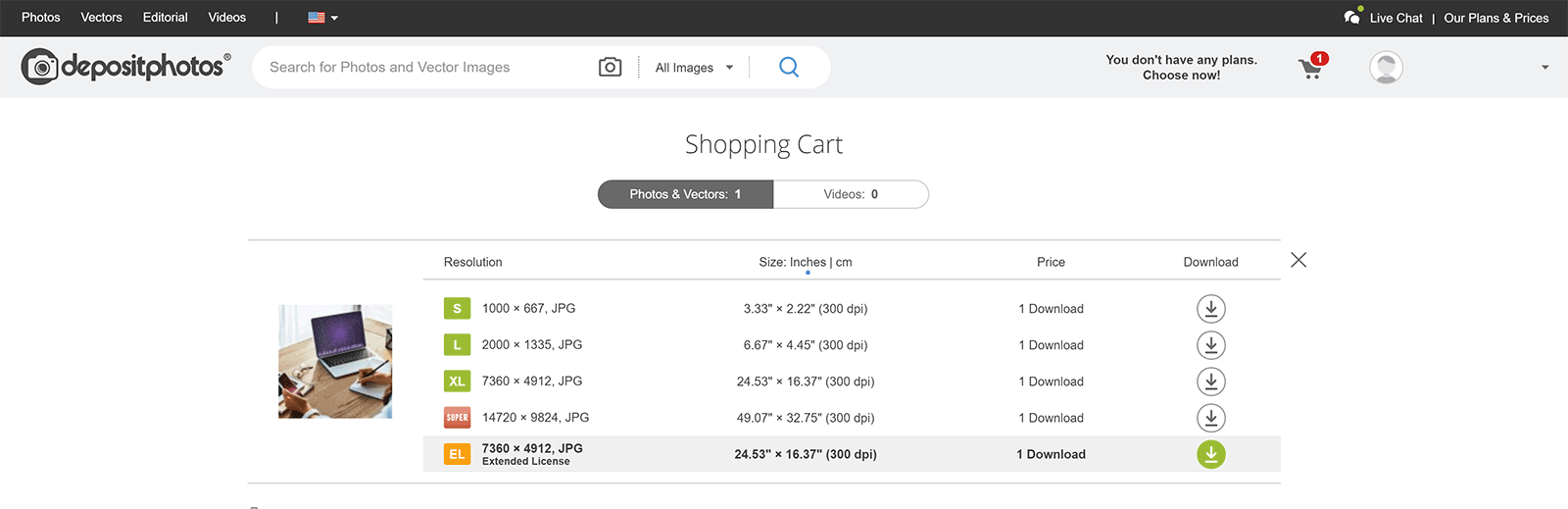This image is a detailed screenshot of the Deposit Photos website, a platform that allows users to search for photos and vector images. Central to the image is a shopping cart icon, with an option to choose the download size of the selected images. The available sizes range from a small 3.33 inches by 2.22 inches to a substantial 24.5 inches by 16.33 inches, showcasing a wide variety in picture dimensions.

On the far left side of the screenshot, there is a depiction of an open laptop computer with a purple screen. A person is seated at a desk in front of this laptop, working with a notepad and paper, suggesting a workspace setup. 

At the top of the screenshot, a black headline bar features several options: "Photos," "Vectors," "Editorial," "Videos," an icon of an American flag with a downward arrow to select the country, a "Live Chat" option, and a link to "Our Plans and Prices." This bar is prominently displayed, indicating the primary navigation tools for users on this website.